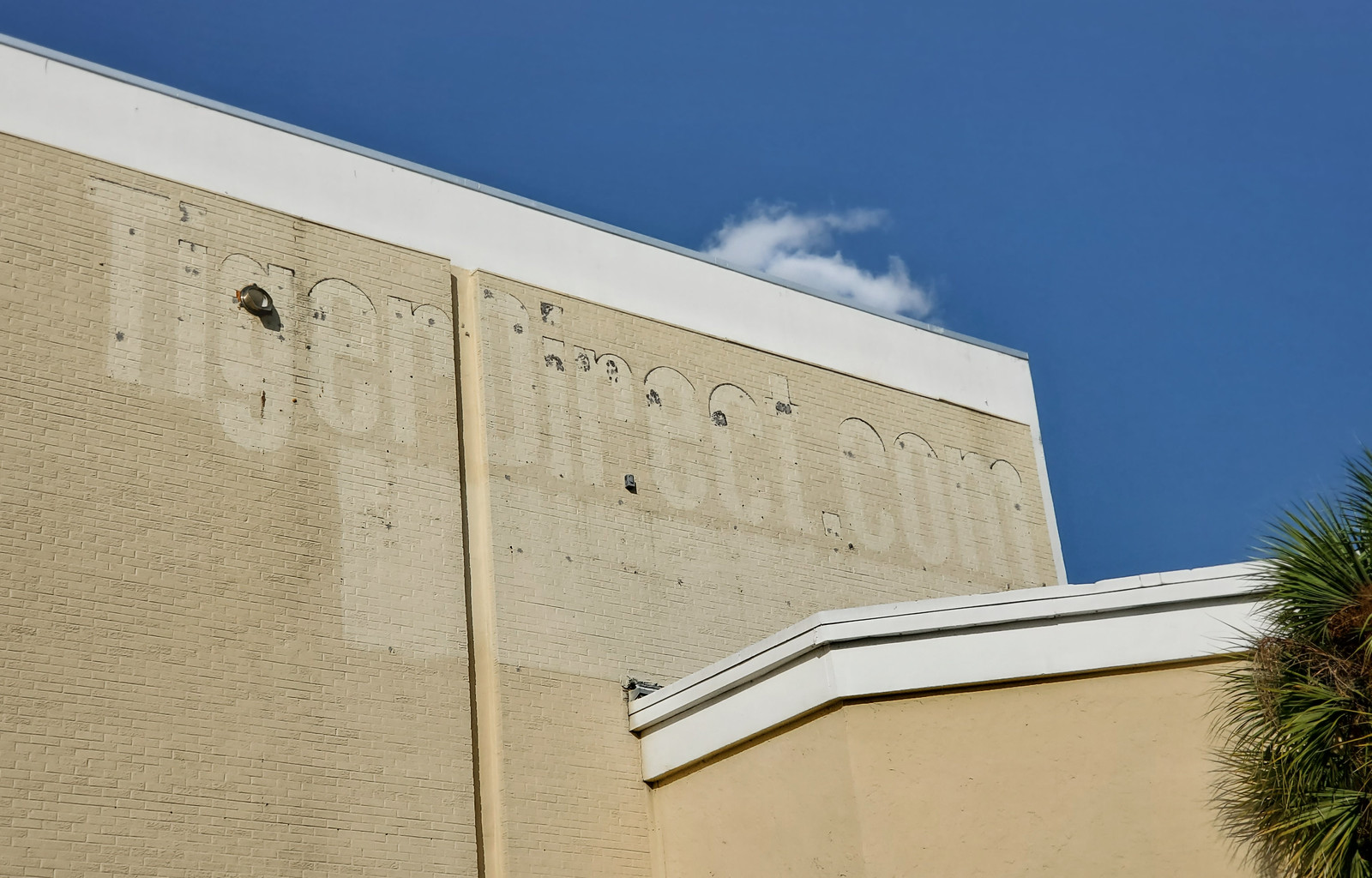In this outdoor image, a vast expanse of vibrant blue sky, accented by a few wispy clouds, dominates the upper portion. Toward the bottom right corner, there are a cluster of tropical trees contributing to the lush atmosphere. The focal point, however, is a prominent beige-colored brick building that occupies the majority of the scene. This building features a distinct white trim along its roofline and a gutter running down its side. The structure is two-storied, with two interconnected parts. Notably, the facade reveals the faint imprint of a sign that once read "TigerDirect.com," just above a lighter rectangular area where an additional sign or banner used to be affixed.